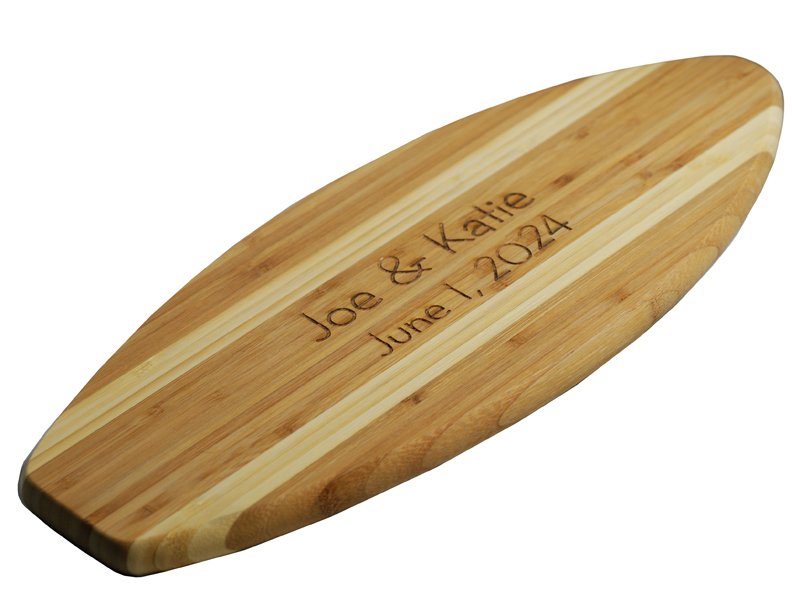The image features a long wooden cutting board shaped like a surfboard, with a light brown surface and lighter beige edges. The design includes two parallel lighter beige lines running along the edges, providing a subtle contrast. In the center of the cutting board, there is a laser-engraved monogram in black that reads "Joe & Katie," with the date "June 1st, 2024" inscribed below it. The board is placed against a white background, highlighting its custom, possibly commemorative design, which could suggest a significant date such as a wedding or anniversary.